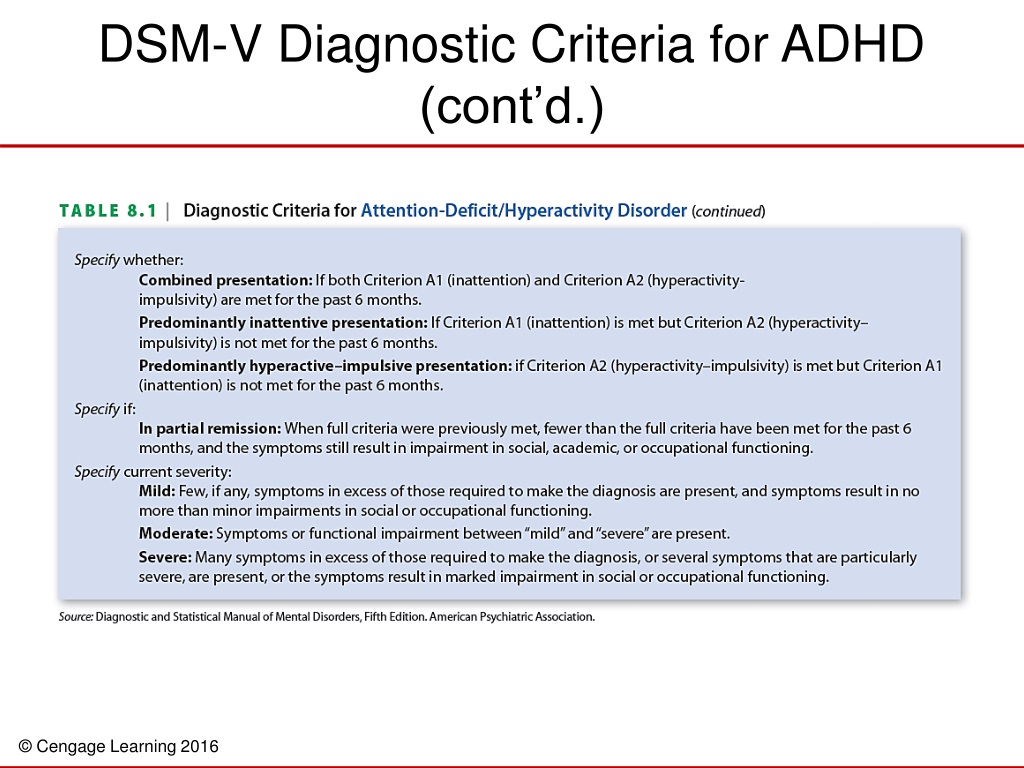The image displays the DSM-V Diagnostic Criteria for ADHD. At the top, there is a heading in bold that reads "DSM-V Diagnostic Criteria for ADHD, Continued." Below this heading, a prominent red horizontal line separates the top section from the content beneath it. Under this line, the text "Table 8.1: Diagnostic Criteria for Attention Deficit Hyperactivity Disorder" is written in green.

Following this description, there is a light blue text box containing detailed criteria for diagnosing ADHD. It outlines the specific presentations based on the criteria met over the past six months. 

Firstly, it specifies the "Combined Presentation," which is applicable if both Criterion A1 (Inattention) and Criterion A2 (Hyperactivity/Impulsivity) are met. 

Next, it describes the "Predominantly Inattentive Presentation," which applies if Criterion A1 (Inattention) is met but Criterion A2 (Hyperactivity/Impulsivity) is not met.

Lastly, it details the "Predominantly Hyperactive-Impulsive Presentation," which applies if Criterion A2 (Hyperactivity/Impulsivity) is met, but Criterion A1 (Inattention) is not met.